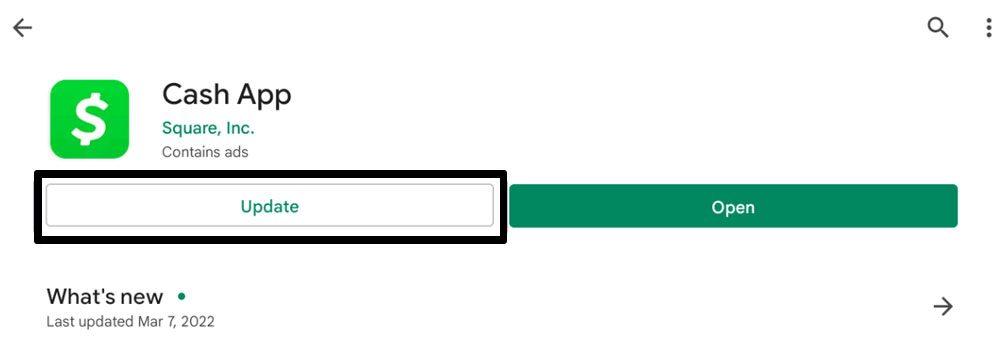The image depicts a screenshot of the Google Play Store interface on a smartphone. At the top of the screen, the app "Cash App" is prominently displayed with its icon, a white money symbol on a green square background, alongside its name. Below the title, "Cash App," the developer is listed as Square Incorporated. 

Two buttons are visible beneath the app's title: "Update" and "Open." The "Update" button is outlined with a black rectangle, while the "Open" button is designed as a solid green rectangle with the text "Open" centered within it. 

Further down, text reads "What's new," followed by "Last updated March 7th, 2022," indicating recent changes to the app. To the top right-hand corner of the screen is a magnifying glass icon, representing the search function within the Play Store. 

This interface reflects a typical prompt users encounter when they need to update an app before opening it.